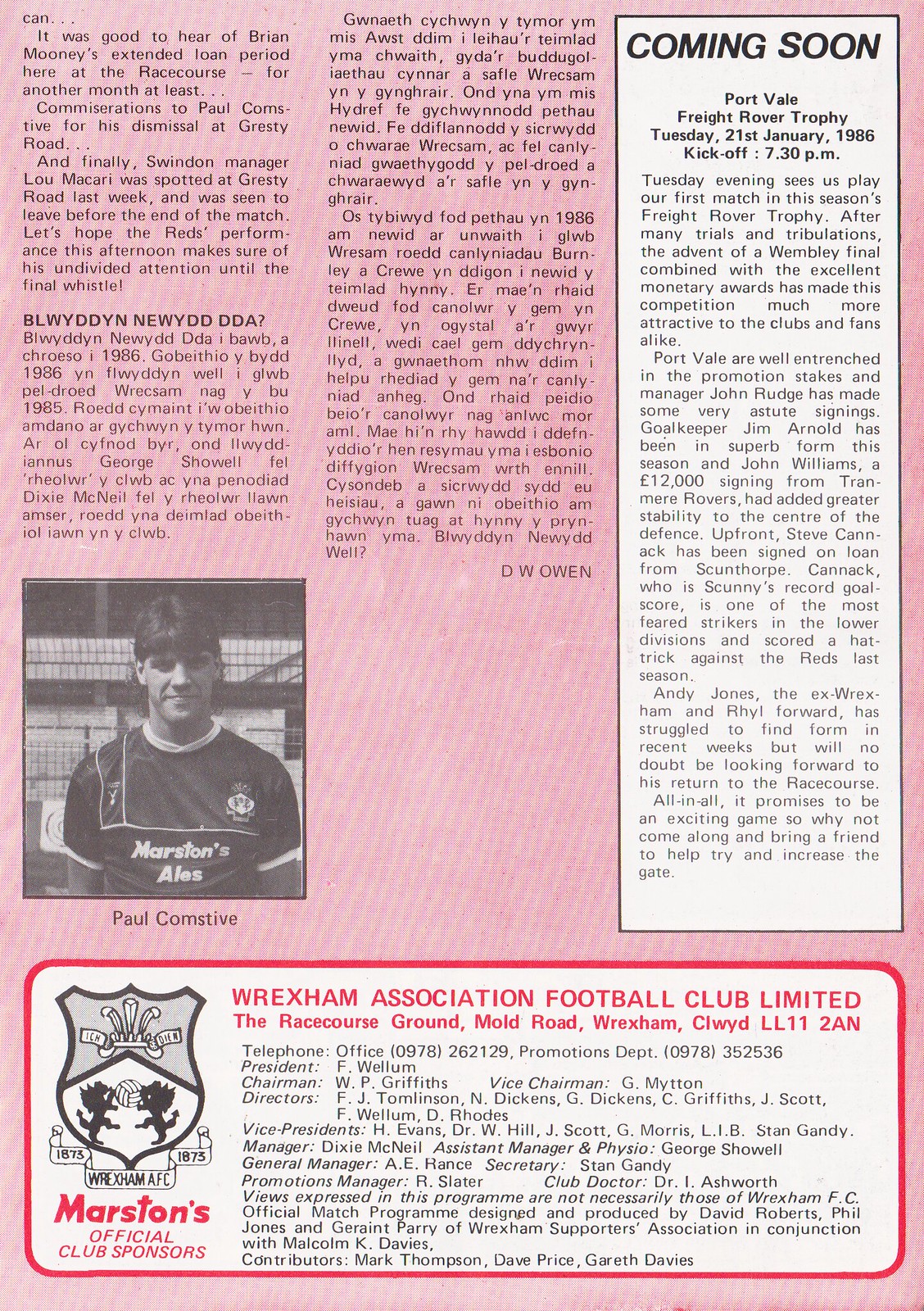The image is a vintage promotional flyer from 1986 for the Wrexham Association Football Club Limited. It features a predominantly pink background with two columns of black and white text dominating the top two-thirds of the page. The right side includes a white inset column announcing an upcoming event: "Coming soon, Port Vale Freight Rover Trophy, Tuesday, 21st January 1986, kickoff 7.30pm." 

Toward the lower-left corner of the page, there's a color photo of a young player named Paul Kornstein, shown from the chest up and wearing a jersey emblazoned with "Marston's Ales." Above the photo, some text appears in a different language. The flyer conveys the excitement around the Freight Rover Trophy, highlighting the significance of the competition with a potential Wembley final and monetary rewards, making it attractive to clubs and fans alike.

At the very bottom, there is a red-bordered rectangle containing an ad for the Wrexham Association Football Club Limited, including contact details, names of the club's president, chairman, directors, vice presidents, manager, general manager, and promotions manager. The Marston's official club sponsors logo, featuring a black and white shield with two facing lions and a flourish, is also included in this ad section. The overall style of the flyer is reminiscent of a printed magazine or newspaper page from the era.